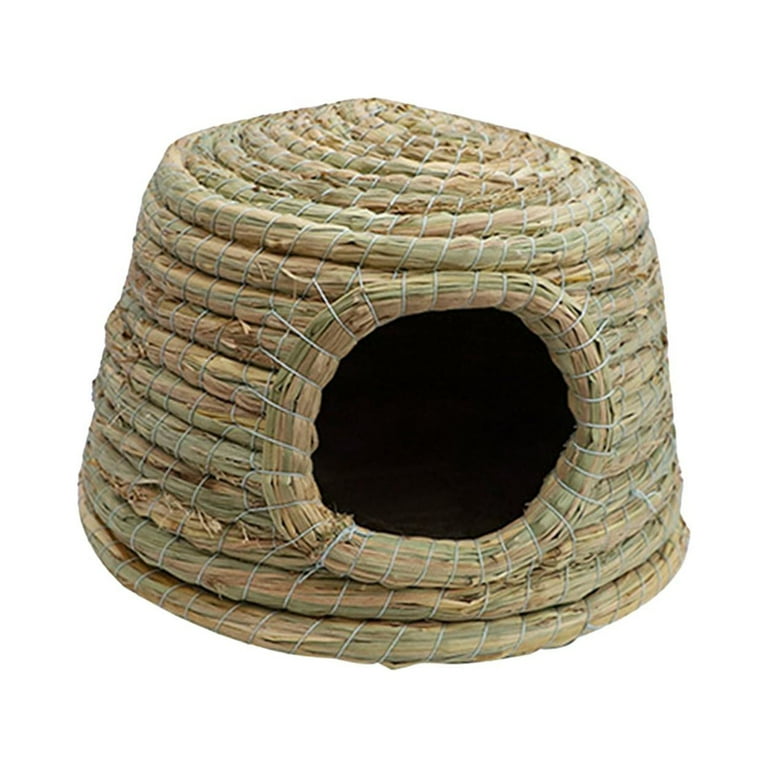This image features a hand-woven pet bed, crafted from a combination of dried and green fibrous twine or wicker-like material. The structure resembles a basket turned upside down, with a distinctive large entrance hole on one side. The hole is bordered by tightly wrapped twine, adding to its organic appearance. The exterior showcases a mix of brown and green colors, indicative of the natural materials used. Set against a plain white background, the interior of the pet bed appears completely dark, lacking any visible cushion or lining. Its overall form suggests a cozy, nest-like space for a cat or dog to curl up inside.